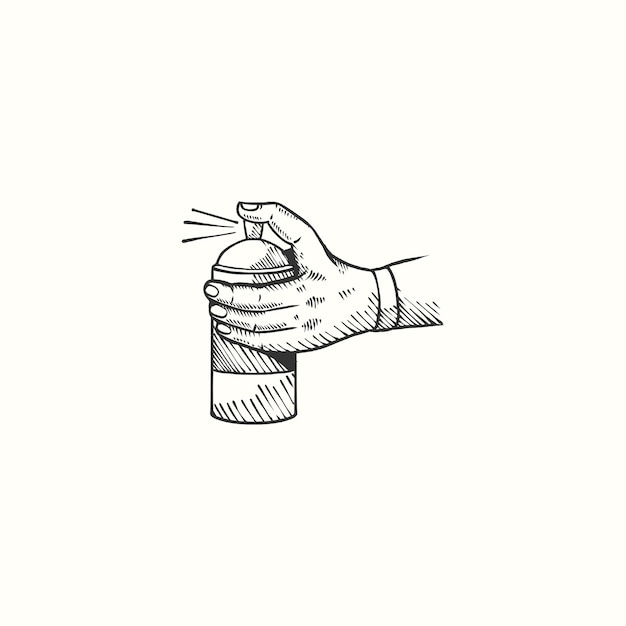A realistic, cartoon-style illustration captures a left hand pressing down on the nozzle of a spray can. The hand's action is evident, with the nozzle visibly being compressed. The can itself is compact, approximately 7 to 8 inches tall and 3 to 4 inches in diameter. The well-groomed fingernails of the person are clearly visible, and their wrist is adorned with a piece of jewelry, adding a touch of personal detail to the image.